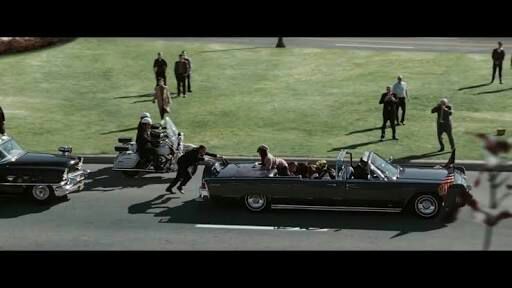The image appears to be a scene from a 1970s film, characterized by its grainy texture and vintage aesthetic. In the foreground, a long black station wagon, typical of the era, is positioned in the left lane of a road. The car's top is down, revealing several passengers inside, with one person notably leaning over the back. Another individual is seen pushing the vehicle from behind, their hands firmly on the car's rear bumper.

Adjacent to this car, there is another sleek, black vintage vehicle partially visible, specifically its front quarter. Between these cars, a cruiser-type motorcycle with two helmeted riders, possibly police officers, is parked, though no distinguishing police insignia or sirens are visible.

A grassy median runs parallel to the road, populated by a group of men dispersed across the area, suggesting a scene of either waiting or gathering. The setting is bathed in daylight, further enhancing the nostalgic ambiance of the captured moment.